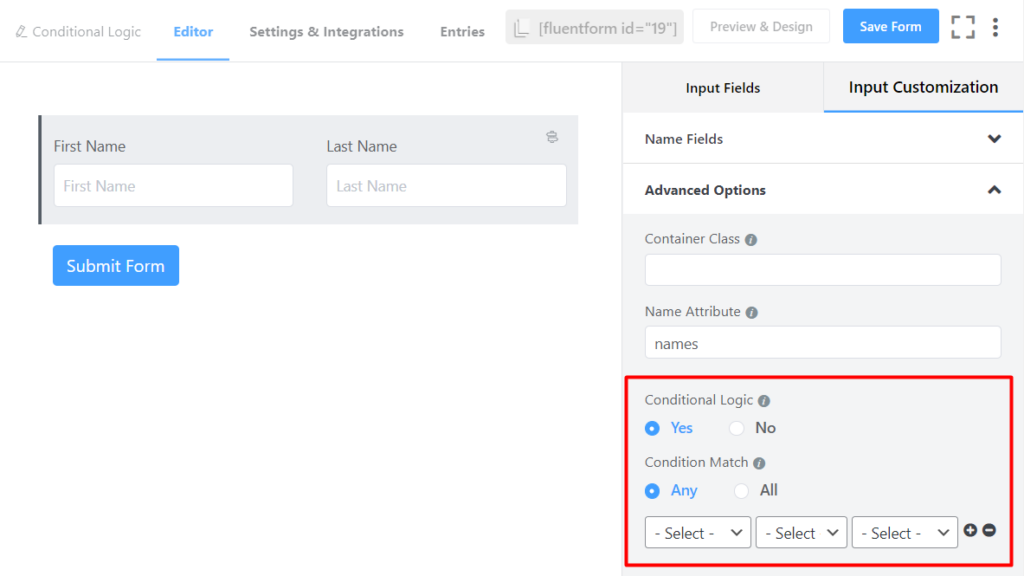This screenshot captures a computer screen displaying a web form interface. The majority of the background is white, interspersed with sections of a gray background. Notably, there are two blue buttons; one labeled "Submit Form" located in the lower left-hand corner, and another labeled "Save Form" positioned in the upper right-hand corner of the screen.

In the lower left-hand corner, a box labeled "Conditional Logic" is visible. This box contains two fields: "Conditional Logic" and "Condition Match," both highlighted with a red rectangular border. Within this area, there are three unselected radio buttons.

At the top of the screen, the interface features several tabs: "Conditional Logic," "Editor," "Settings," "Integrations," "Entries," "Preview," and "Design." There are also fields for "First Name" and "Last Name," though specific entries in these fields are not detailed in the caption.